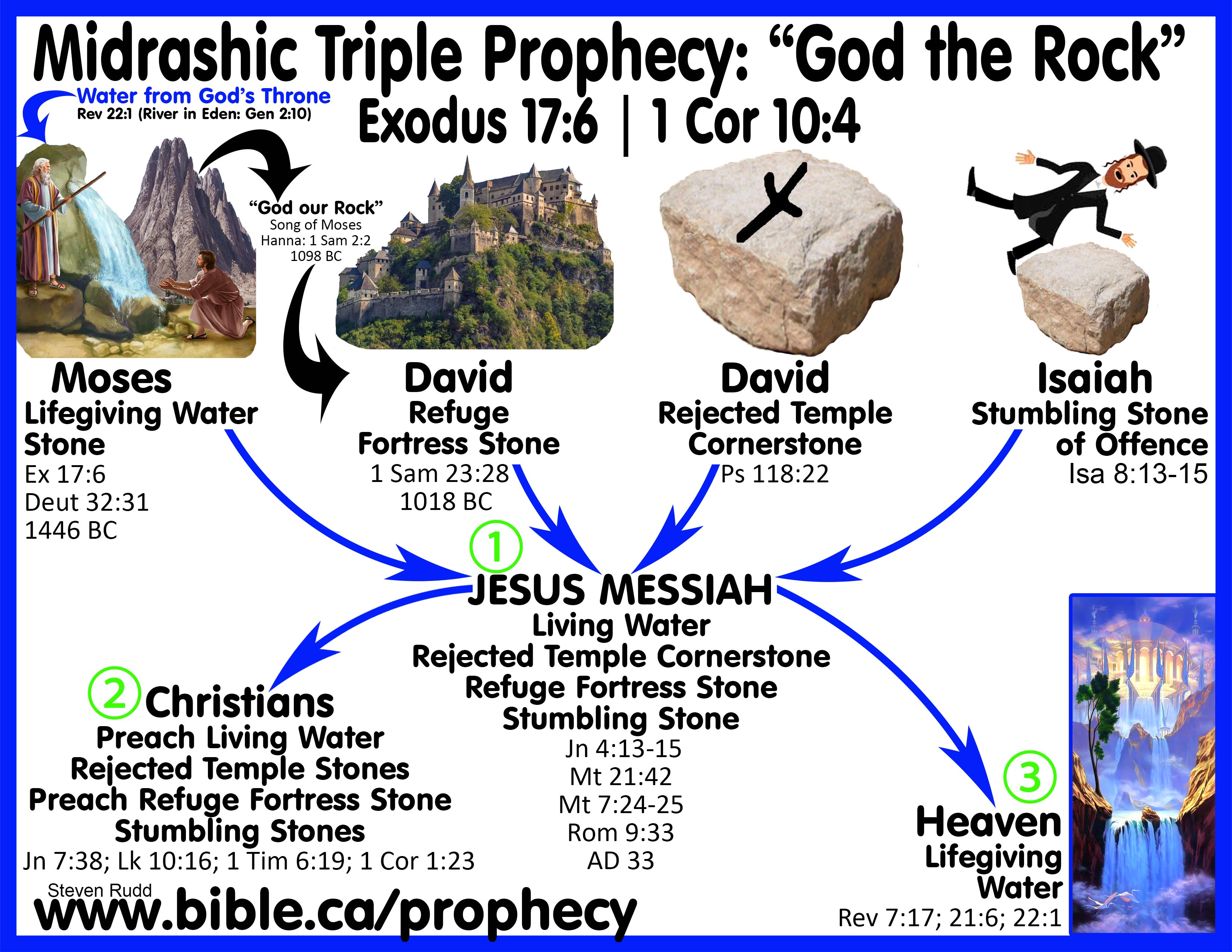The image is a horizontally oriented religious infographic bordered in royal blue. The background is white and features bold black text. At the top, it reads "Midrashic Triple Prophecy: 'God the Rock'". Below this, key biblical references are highlighted, including Exodus 17:6 and 1 Corinthians 10:4. 

The infographic includes a series of images with accompanying biblical scenes and prophecies:
1. On the left, an image labeled "Moses, life-giving water stone" from Exodus 17:6 (1446 B.C.), depicts Moses by a rock with water flowing from it and another figure kneeling below.
2. Next, an image of a castle labeled "David, refuge fortress stone" (1018 B.C.) indicates a biblical scene from Samuel.
3. Following this is a stone with a cross, labeled "David, rejected temple cornerstone."
4. The final image in this row is labeled "Isaiah, stumbling stone of offense," featuring a stone beside a figure symbolizing Isaiah.

In the center of the image, arrows from these scenes converge on a depiction of Jesus, labeled "Jesus, Messiah: Living Water, Rejected Temple Cornerstone, Refuge Fortress Stone, Stumbling Stone" (A.D. 33). Additional Bible verses are referenced here, emphasizing Jesus' fulfillment of these prophecies.

Arrows lead from Jesus to:
- Green-labeled section (1): "Christians: preach living water, rejected temple stones, refuge fortress stone, stumbling stones."
- Blue-labeled section (2): "Heaven: life-giving water" depicted by a waterfall and sky.

In the bottom corners of the image, text attributes the graphic to Stephen Rudd and provides a link: www.bible.ca/prophecy.

This comprehensive visual guide illustrates the prophecy connections between Moses, David, Isaiah, and Jesus, and how Christians and the promise of Heaven are intertwined within biblical scripture.